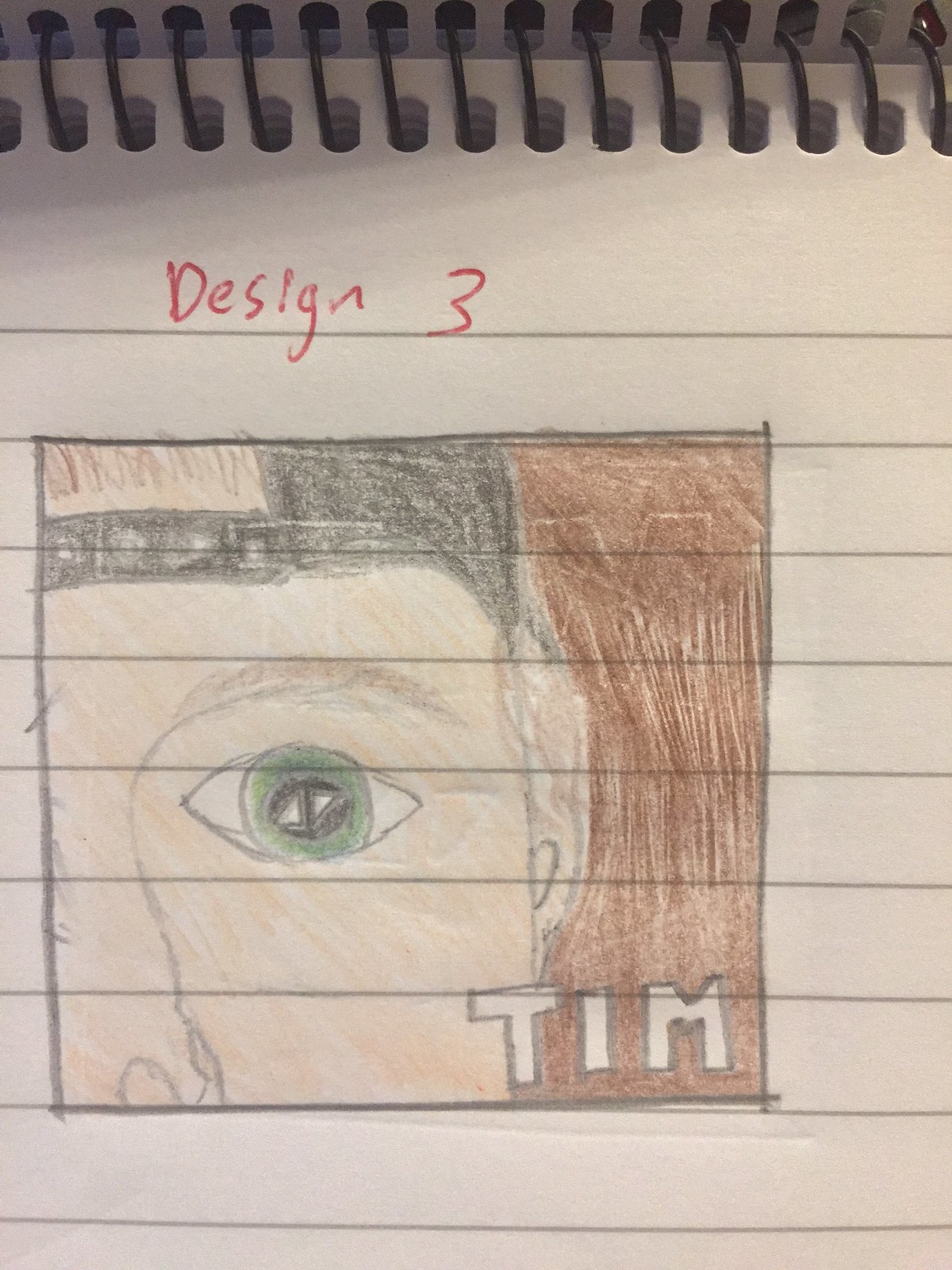In this amateur photo, a lined notebook sheet is prominently featured with the metal rings of the notebook visible at the top. The first line, meant for headings, reads "Design 3" in bold red capital letters. Below this heading, there is a comic-like illustration drawn in pencil crayon. The sketch, positioned on the upper left, depicts the partial face of an individual wearing a black baseball cap turned backwards. The details include a green eye, a single eyelash, and half a nose, where the image cuts off before reaching the mouth. There is a brown section in the background with the name "Tim" written in bold, uppercase letters. A faint, initially attempted "Tim" can be seen underneath, partially erased and the letters drawn over.